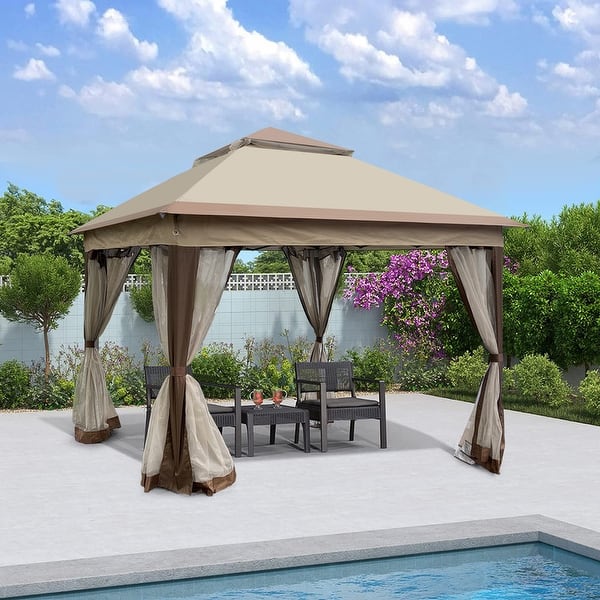The image depicts an inviting poolside scene featuring a stylish cabana. In the foreground, a corner of the pool showcases clear, turquoise water, contrasting beautifully with the smooth, light gray ground encircling it. The central focus is a neat, square-shaped cabana, distinguished by its beige-gray canopy roof and sturdy brown poles at each corner. Beige curtains, tied midway, hang gracefully from these poles, framing the cozy space within. Inside the cabana, two black patio chairs flank a small side table adorned with two glasses of drinks, offering a perfect spot for relaxation. Behind the cabana, a blend of lush green bushes and vibrant purple flowers form a picturesque backdrop, while a gated wall delineates the boundary. Above, the sky is a serene blue, dotted with light, fluffy clouds, completing this tranquil outdoor setting.